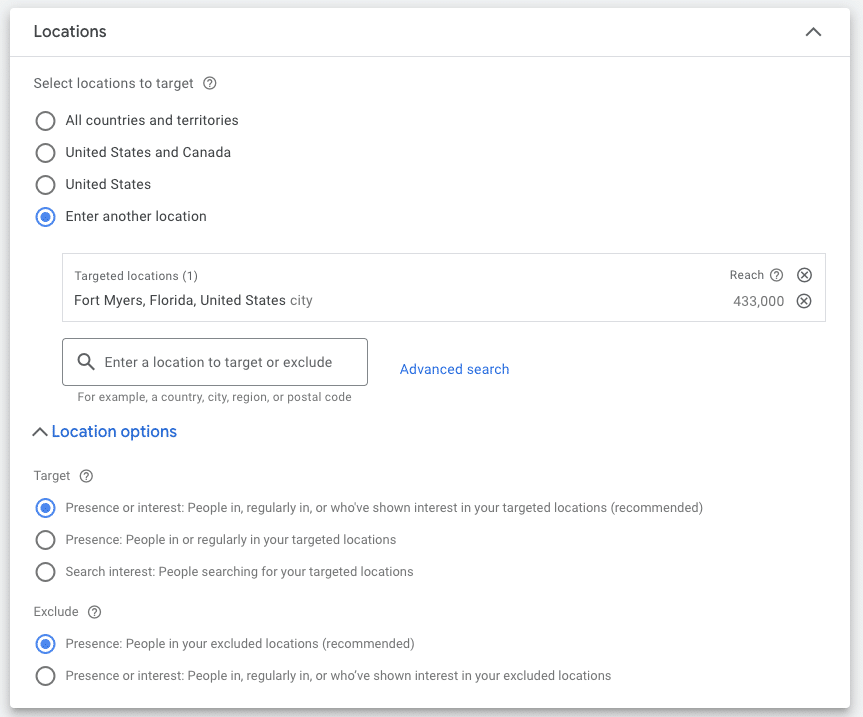The image displays a geographic targeting interface commonly used in advertising or data analytics. Users are able to select specific locations to target or exclude from their campaign. In this instance, the United States and Canada are not selected as targets. Further, additional parameters allow for refined targeting, such as targeting people who are either currently in, regularly visit, or show interest in specified locations—though some of these options are currently unchecked. The image indicates that Fort Myers, Florida, with an audience reach of 433,000, is the chosen targeted location. There are advanced search options available to further tailor the targeting criteria, including the ability to exclude people in certain areas. The recommended settings for including 'presence or interest' of people in the targeted locations and excluding 'presence' of people in excluded locations are checked.